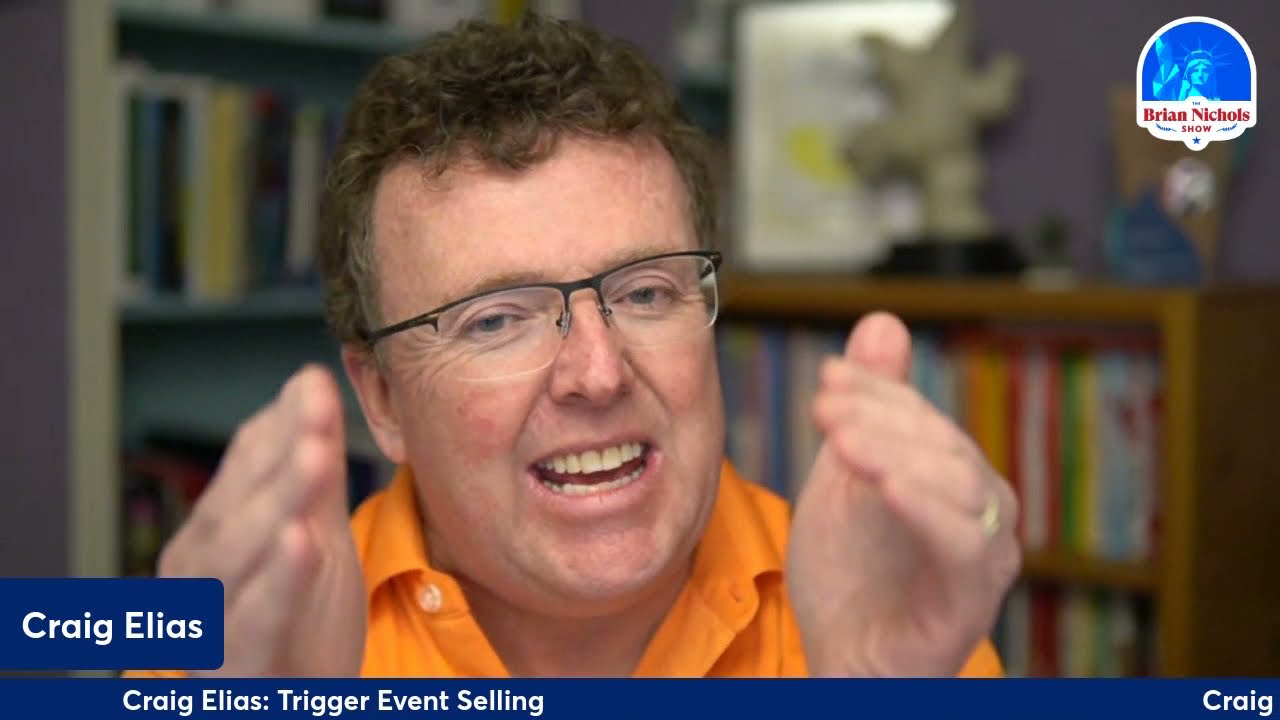In this image, we see a highly animated man named Craig Elias, captured in mid-gesture with his hands raised near either side of his face, head slightly tilted as he speaks energetically. He is wearing a bright orange short-sleeved shirt, sporting brown curly hair, and glasses. There is a ring visible on one of his hands. The background is a blurred bookshelf, suggesting he might be sitting in a library or a home office. The screen displays his name, "Craig Elias," prominently in white text on a blue background in the lower left and bottom borders, with the phrase "Trigger Event Selling" accompanying his name. Additionally, the lower right corner of the screen also has his name, "Craig." The upper right features the logo for "The Brian Nichols Show," indicating that Craig Elias is likely a guest on this show, discussing the concept of trigger event selling. The dynamic pose and lively expression suggest he is passionately involved in explaining his viewpoint during this vlog, streaming show, or TV segment.